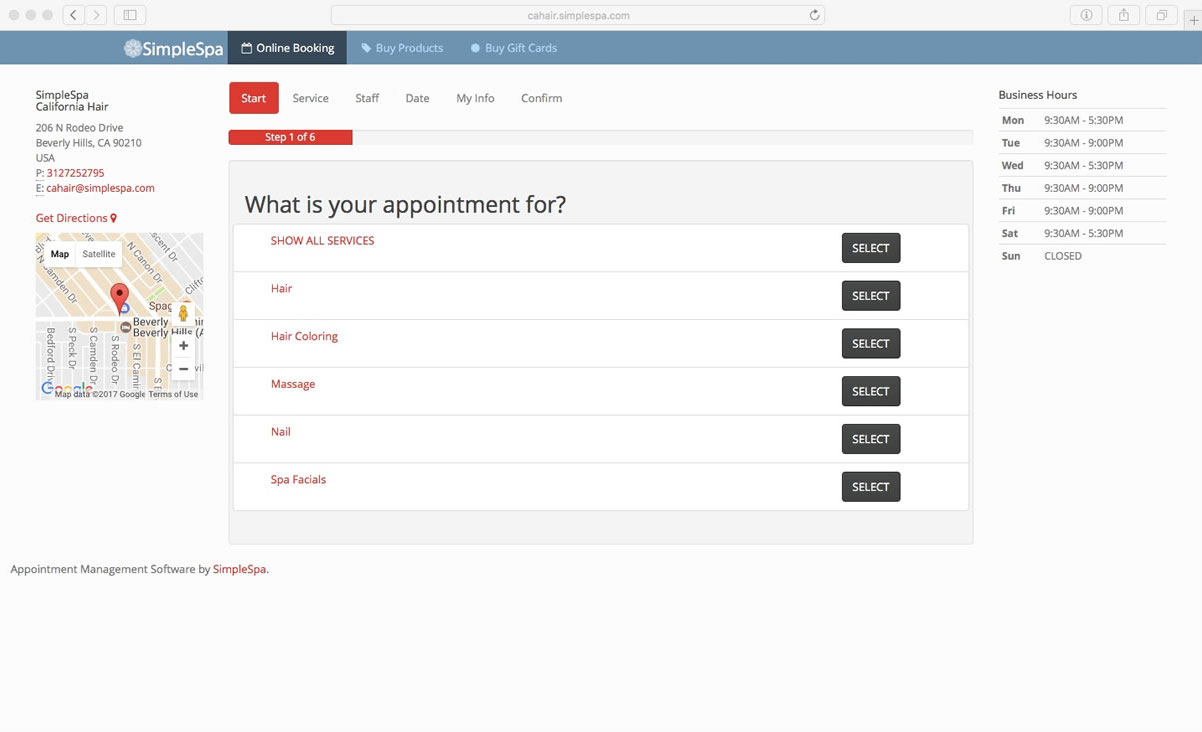A detailed image caption for a website called Simple Spa:

The image depicts the booking page of Simple Spa's website, accessible at kahairsimplespa.com. The top of the page features a tan-gray address bar containing the URL. Just below, a light blue navigation bar prominently displays "Simple Spa" in white text on the left. Adjacent to the spa’s name are navigation options: "Online Booking," "Buy Products," and "Buy Gift Cards," all in white font. 

Beneath the navigation bar, black and gray text provides step-by-step booking instructions. The left side indicates "Start," followed by tabs labeled "Service," "Staff," "Date," "MyInfo," and "Confirm" in sequence. A red text indicates the user is on "Step 1 of 6."

Below, a gray bar serves as a separator, leading to the section titled "What is Your Appointment For?" Here, options are presented for various services, including "Show All Services," "Hair," "Hair Coloring," "Massage," "Nail," and "Spa Facials." Each service category is accompanied by a series of black buttons labeled "Select" in white, enabling users to specify their desired salon services.